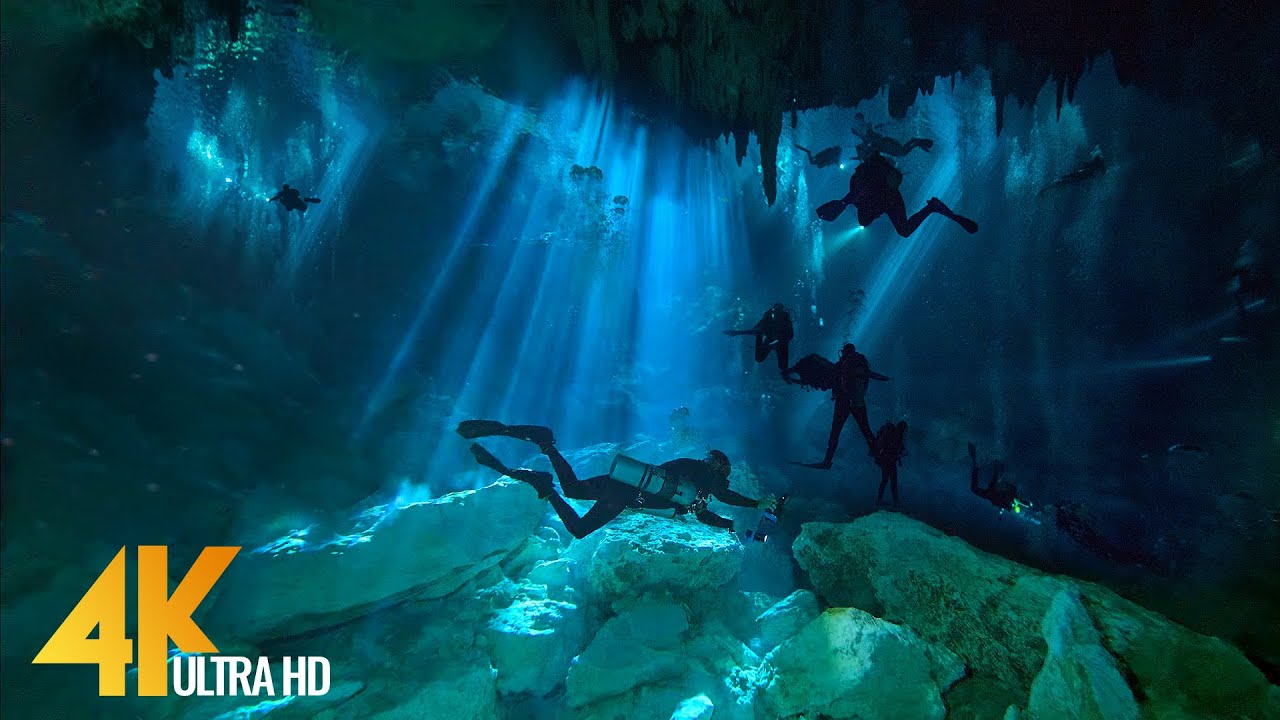The image shows a surreal underwater cave diving scene, possibly a frame from a video or documentary. In the crystal blue water, illuminated by penetrating rays of light from above, at least 13 scuba divers with professional gear and oxygen tanks are seen. The majority are in the middle of the image, with one diver hanging in the top left. The divers appear silhouetted against the beams of light, which cluster around the center, highlighting the long, large, light-colored rocks scattered on the cave floor. One diver in the foreground holds a flashlight with both hands. On the bottom left, there's a logo reading "4K" in yellow-orange letters and "Ultra HD" in white, enhancing the high-definition visual appeal of the scene.